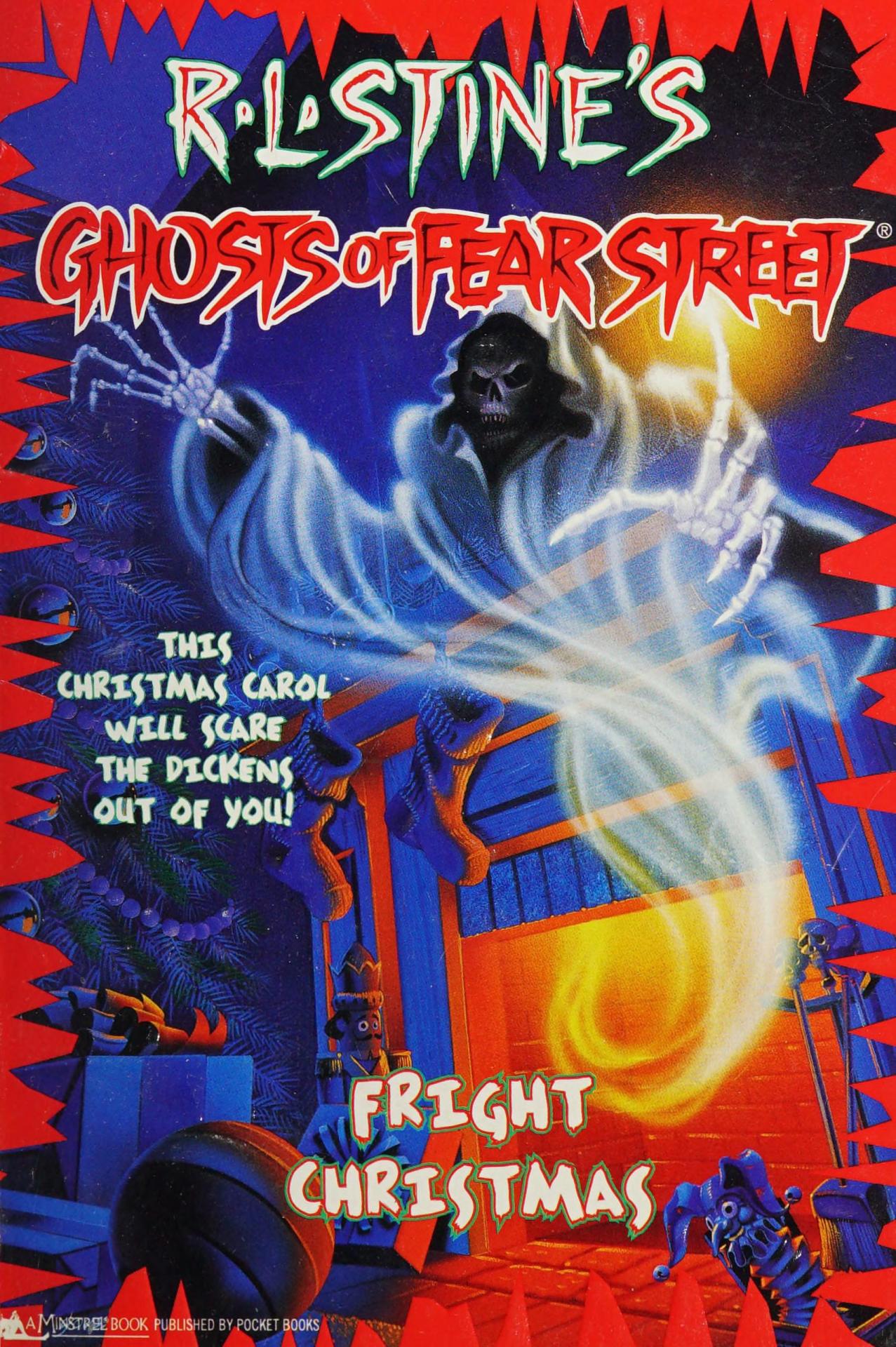The image depicts a Halloween-themed comic book cover, adorned with striking visual elements. The borders of the page feature rows of triangular, red spikes, enhancing its eerie aesthetic. Dominating the center is an illustration set against a dark, blue-toned background, suggesting a nighttime scene. Emerging from what appears to be a garage door is a ghostly figure reminiscent of the Grim Reaper, but with a dusty, translucent appearance. Only the skeletal face and hands of this specter are visible, adding to its haunting presence. Below, additional menacing characters inhabit the scene, intensifying the overall atmosphere of dread. The title "R.L. Stine’s Ghosts of Fear Street" appears prominently in bold, red letters. The cover also teases, "This Christmas Carol Will Scare the Dickens Out of You," while the subtitle "Fright Christmas" is inscribed at the bottom in white lettering.